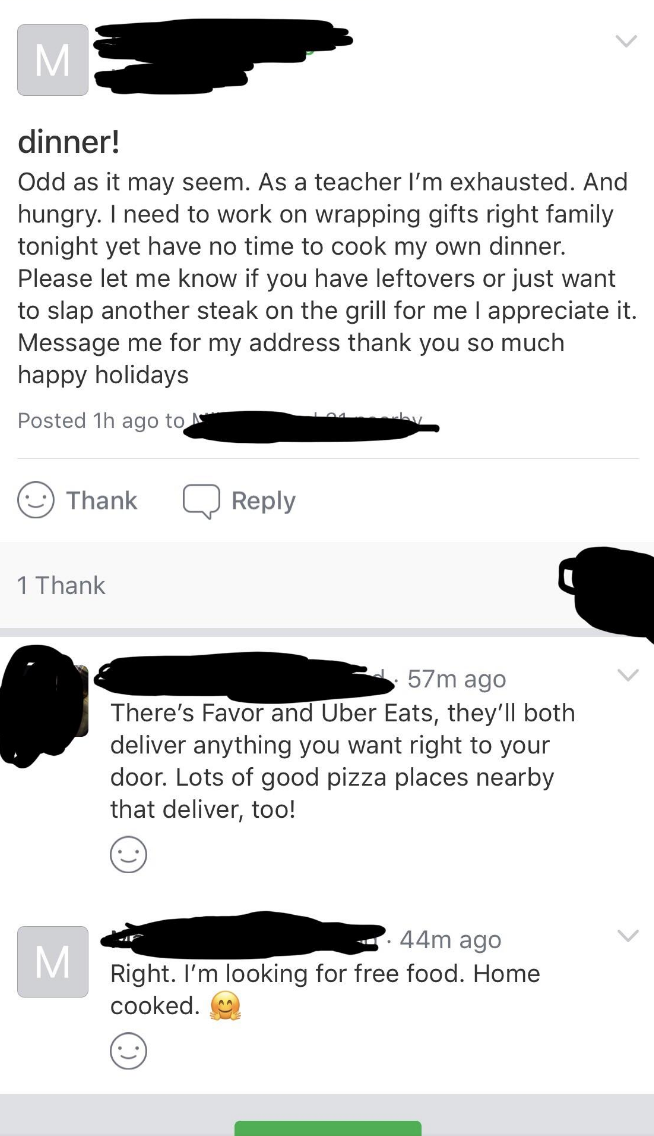This image features a social media post and subsequent comments, partially anonymized for privacy. At the top, a user with a profile picture of a gray square with an "M" initially posts, saying: 

"Dinner. Odd as it may seem, as a teacher, I'm exhausted and hungry. I need to work on wrapping gifts, write family tonight, yet have no time to cook my own dinner. Please let me know if you have leftovers or just want to slap another steak on the grill for me. I appreciate it. Message me for my address. Thank you so much. Happy Holidays."

This post was made an hour ago, with some parts covered by a black highlighter. Below the post, there are two interactive options labeled "Think" and "Reply."

The first comment, made 57 minutes ago, offers a solution: 

"There's Favor and Uber Eats. They'll both deliver anything you want right to your door. Lots of good pizza places nearby that deliver, too!"

Responding to the first comment, the original poster replies with a lighthearted note:

"Right, I'm looking for free food, home-cooked. 😊"

The bottom section of the image features a light gray rectangular banner extending from one side to the other, with a green horizontal bar centered at the very bottom. All names and timestamps below the initial post are crossed out to maintain anonymity.